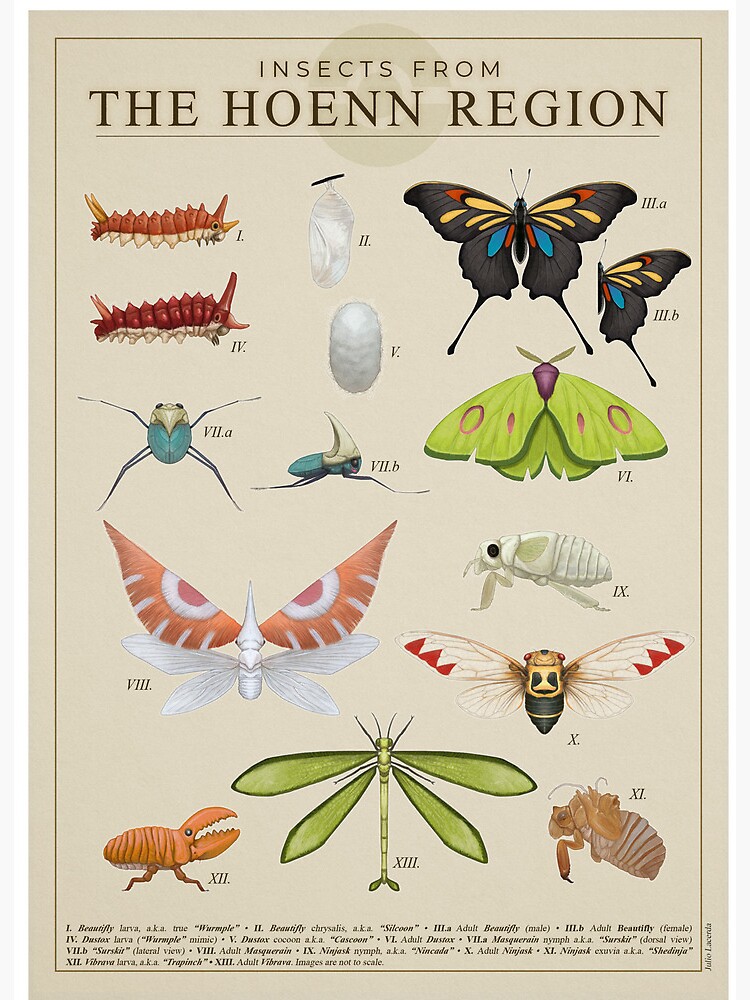This image is an informational graphic showcasing a variety of colorful insects from the Hoenn region. The title at the top reads "Insects from the Hoenn region." The illustrations, rendered in a vibrant, cartoon-like style, include spiky red caterpillars and white cocoons. To the right, you'll find black butterflies adorned with striking yellow, blue, and red circular patterns. Among the diverse creatures are blue beetles and a bright green moth that features distinctive purple circle patterns on its wings. Additional illustrations include various moths, flies, cicadas, a flea-like water bug, and a green dragonfly. The poster, though detailed, has small, unreadable text at the bottom, completing this vividly animated entomological catalog.